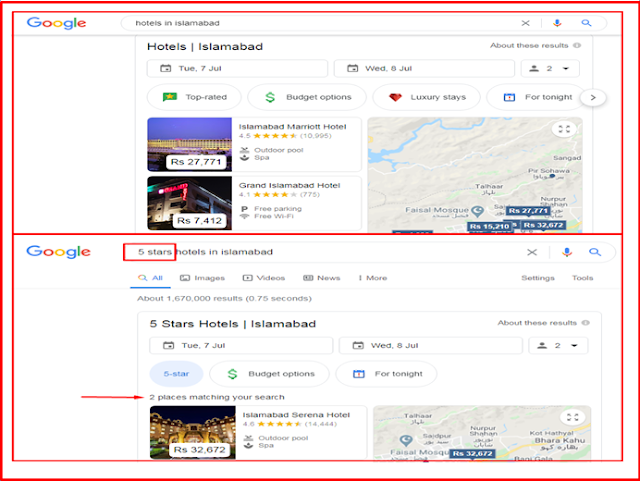The image showcases two Google search results pages, presented side by side, each bordered and separated by prominent red strips. The left page displays a search query for "hotels in Islamabad," while the right page shows a refined search for "five-star hotels in Islamabad." Both search result pages highlight various hotel options in the city, with snippets of descriptive text and filter categories visible. On the left side, phrases like "top rated," "budget options," and "luxury stays for tonight" can be spotted among the results. In the search results, notable establishments such as the Islamabad Serena Hotel, the Islamabad Marriott Hotel, and the Grand Islamabad Hotel are listed. The interface also includes tabs for different types of search results categories, such as "All," "Images," "Videos," "News," and an additional tab that is not fully visible in the image.